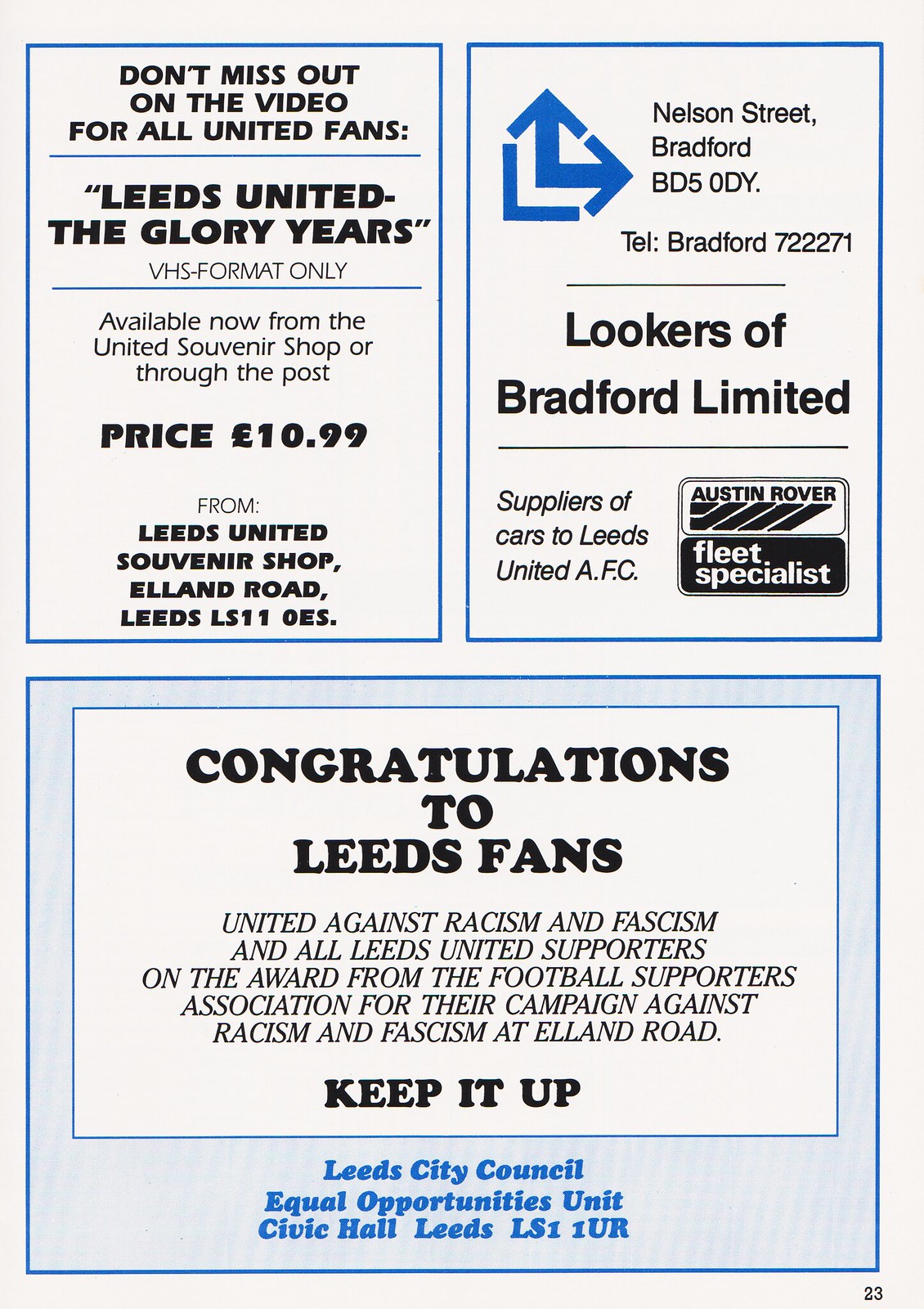The image features three advertisement blocks, all outlined in blue. The block on the top left promotes a VHS tape titled "Leeds United: The Glory Years," exclusively available for $10.99 at the United Souvenir Shop or through the post. The block on the top right details an advertisement for Lookers of Bradford Limited, located on Nelson Street, Bradford. It includes their telephone number, 722271, and highlights their role as suppliers of cars to Leeds United AFC, showcasing a black and white Austin Rover Fleet Specialist logo. The substantial block at the bottom congratulates Leeds United fans for their campaign against racism and fascism at Elland Road, a recognition awarded by the Football Supporters Association. It encourages supporters to "keep it up," and acknowledges support from Leeds City Council's Equal Opportunities Unit.